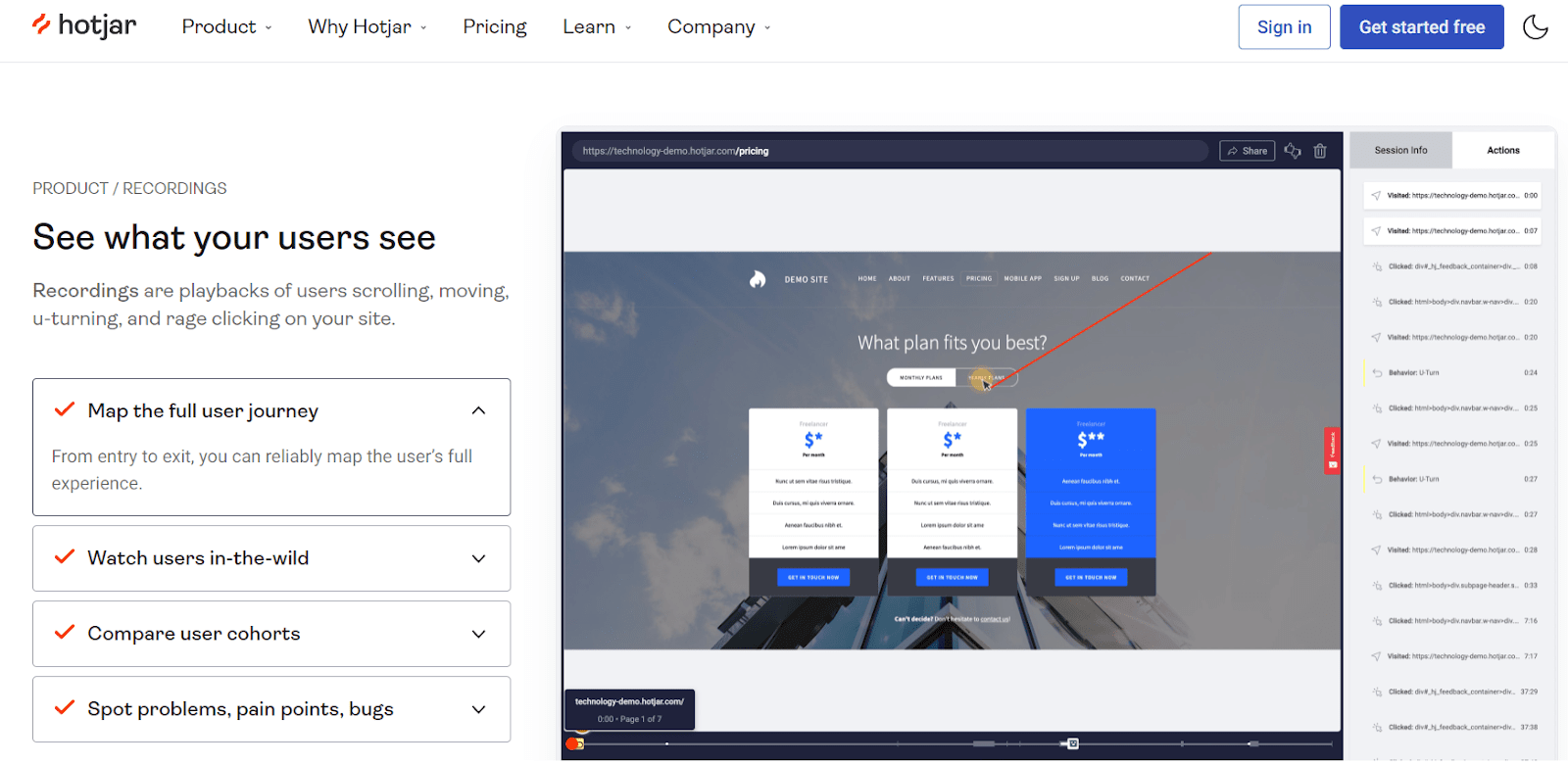Here is the detailed and cleaned-up caption for the image:

---

The image is from a website, set against a white background. In the upper left-hand corner, the word "Hotjar" is displayed in black. To the right, several black text links are sequentially listed: "Product," "Why Hotjar?," "Pricing," "Learn," and "Company."

On the upper right-hand side of the page, there is a white bar with the blue text "Sign in." Just below, a blue button with white text says "Get Started Free," accompanied by an icon resembling a half moon.

Below this, on the left side of the page, there is a section labeled "Products / Recordings" in black text. Under this header, the text "See what your users see" appears in black, followed by a description: "Recordings are playbacks of users scrolling, moving, U-turning, and rage-clicking on your site." Additionally, four clickable boxes are listed vertically, each featuring a red checkmark on the left side and black text on the right. They read as follows:
1. "Map the full user journey from entry to exit. You can reliably map the user's full experience."
2. "Watch users in the wild."
3. "Compare user cohorts."
4. "Spot problems, pain points, bugs."

To the right of this section is a striking image depicting a skyscape with a tall skyscraper, viewed from the ground looking upwards. Overlaying this image are two white boxes positioned on the left and a blue box on the right, with white text across the top stating "What plans fit you best."

Further to the right, there is another box, albeit partially blurred and difficult to decipher. This box features a gray section on the left and a white section on the right, with sixteen lines of text listed below, which are not legible in the image.